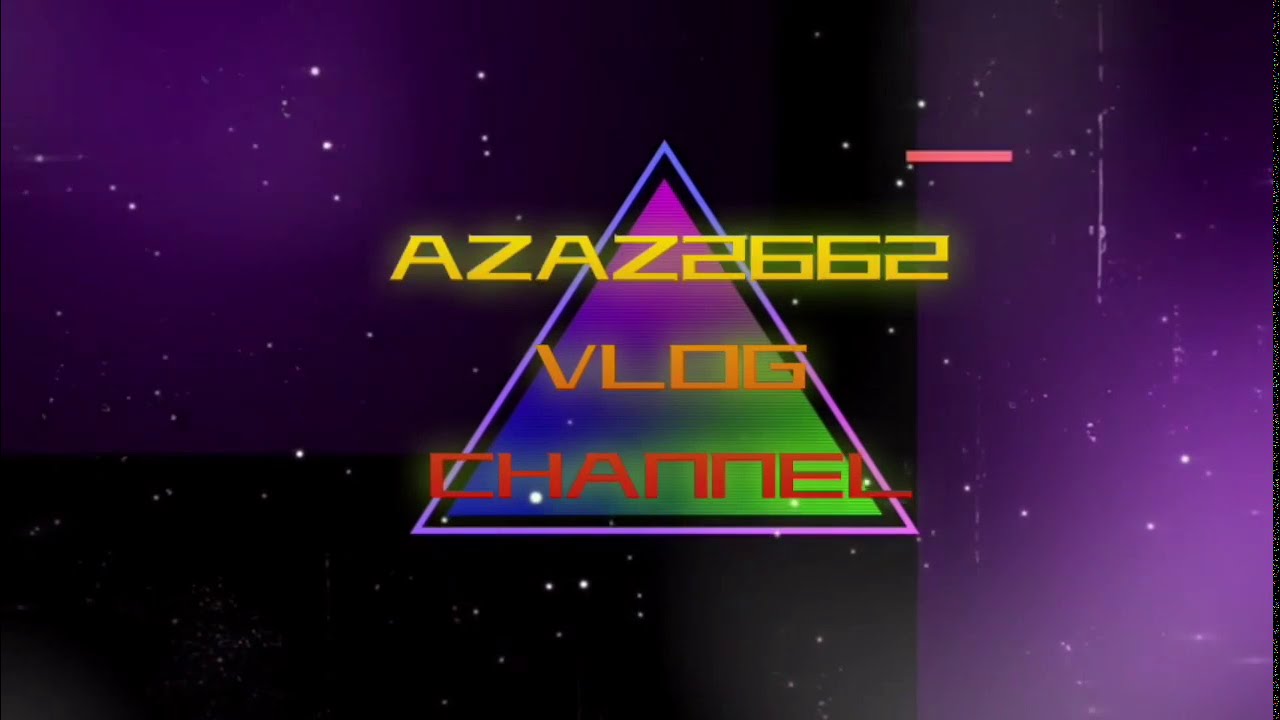The image is a graphical design with an outer space theme, featuring a predominantly black background dotted with small white stars. A hazy purple effect appears in two separate areas: a vertical rectangle along the right edge, and an amorphous shape in the upper left corner. Central to the image is an equilateral triangle, which is colorfully gradiented—green in the bottom right corner, blue in the bottom left, and purple at the top. The triangle is bordered first by a black outline, then a light blue one. Superimposed on this triangle in bold, yellow text is "AZAZ2662" at the top, followed by "Vlog" in yellow, and "Channel" in orange, creating a striking focal point for what appears to be a YouTube banner.